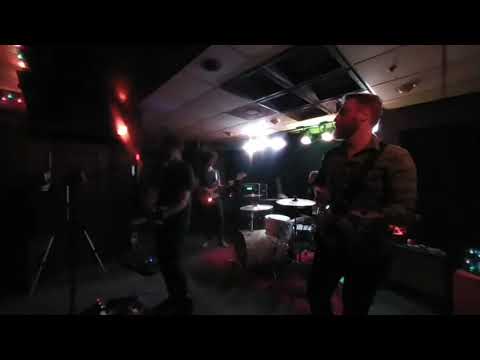This horizontally rectangular, full-color photograph captures a dimly lit indoor performance by a band, likely in a bar or a small venue. The image features a black border only at the top and bottom. The ceiling consists of low white panels with sparse lighting, primarily originating from the back of the stage. The room has a predominantly dark ambiance, punctuated by white and red lights that reflect off various objects within the space. 

In the foreground, one can discern a Caucasian male with short light hair, a full mustache, and a beard. He is wearing dark pants and a long-sleeved, collared shirt. He stands at the front of the stage, presumably singing, but the low lighting obscures many of his details. To his right, another guitarist is similarly poorly lit, making his instrument hard to see, but he appears to be wearing similar dark attire. 

A white drum set is visible in the background, illuminated by spotlights from above. Although the drummer is not visible, the lights highlight the drum area significantly. To the left of the drummer, another figure dressed in black is playing a guitar, possibly a bass. Red lights on the left side of the room add a subtle glow to the scene.